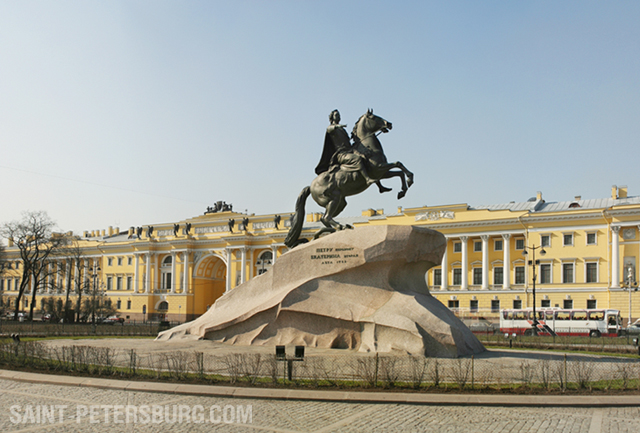The photograph captures a striking bronze statue in a city plaza. At the bottom left corner, the image is marked with "st-petersburg.com" in white text. The monument is set on a large, asymmetrical stone base that rises like a small hill. Atop this stone stands a dynamic statue of a horse rearing on its hind legs, with its front legs raised into the air. Mounted on the horse is a caped man with neck-length hair, his right arm outstretched, pointing to the right. 

In the background, a grand yellow building spans the width of the image, featuring multiple windows, white columns, and an archway that serves as an entrance. Trees with sparse foliage and lampposts are positioned in front of the building, contributing to the stately ambiance. A concrete walkway encircles the monument, bordered by patches of grass and small shrubs. To the right of the monument, an older-style white bus with red detailing moves along a road in front of the building. Overhead, the sky is clear and blue, suggesting a sunny day.